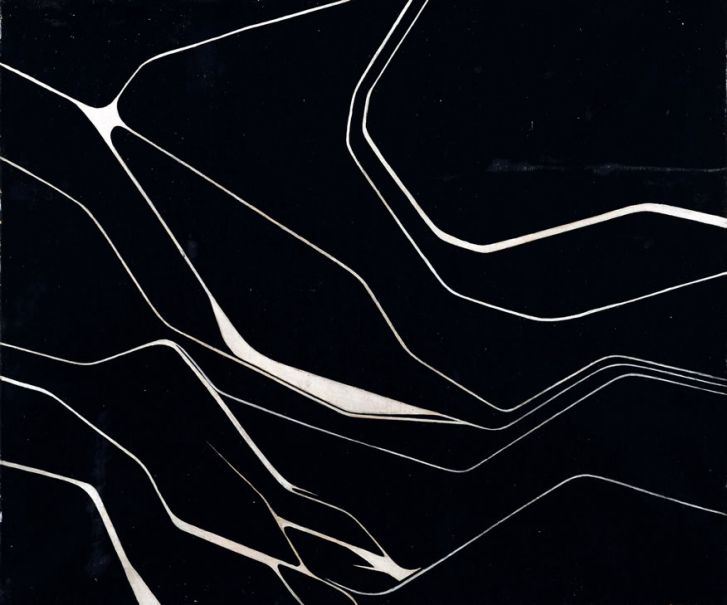The image is a stark black and white illustration with a dominant black background that is crisscrossed by intricate white lines and cracks. These white lines form a web-like structure, resembling veins or the texture of a marble but with a more rigid and structural appearance. They start from the left and branch out towards the right, occasionally curving up or down, creating various thicknesses and patterns. In the upper right, the lines cluster to suggest the appearance of stones or rocks, with some lines creating the visual effect of one rock resting on another. There is a patch of white in the upper left that mimics the effect of light shining through. This radiating white area is echoed by a similar but smaller white patch underneath it in the middle of the image. The overall effect is reminiscent of looking up from a dark hole, with faint light seeping in through the cracks above. Additional white lines are scattered towards the bottom and left, varying in thickness and giving the impression of a natural, uneven fracture pattern. The composition as a whole conveys a sense of depth and rugged texture through its stark black and white contrast.